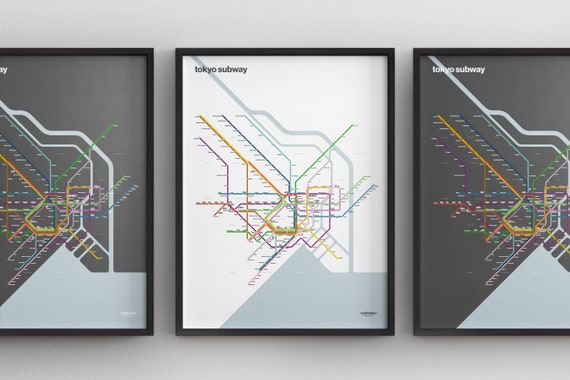The image is a horizontal rectangular composition featuring three framed diagrams of the Tokyo Subway system against a grey, gradient background that darkens towards the bottom. Each diagram is encased in a sleek black frame, with the central drawing fully visible and the two flanking ones slightly truncated. The centerpiece map is set on a white background with the text "Tokyo Subway" in black, illustrating a dense network of streets and different coloured subway lines, including orange, yellow, green, blue, purple, turquoise, and red. The maps on either side, which may also represent Tokyo, feature grey backgrounds with white "Tokyo Subway" text. These diagrams highlight different subway routes in various colors, though some textual details and features, particularly in the bottom right corner, remain too small to decipher.